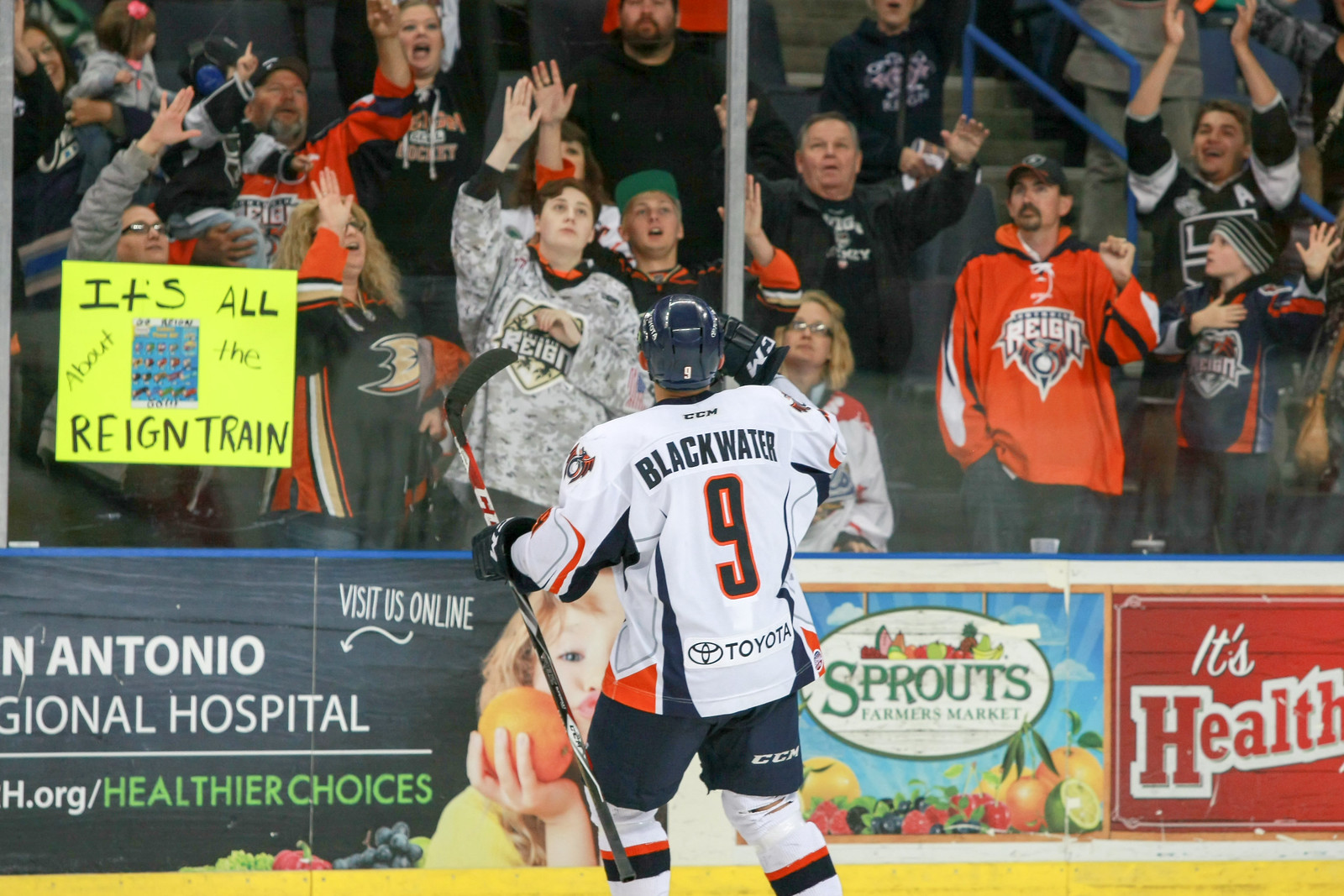A thrilling moment captured from an intense hockey game featuring the Ontario Reign. Player Blackwater, donning the number nine jersey, is in action. His white jersey is accented with striking hues of orange and blue, accompanied by a blue helmet. The atmosphere in the arena is electric, with numerous fans in the stands enthusiastically raising their arms and banging on the glass. A prominent Toyota advertisement is visible at the bottom of the display. To the left, a vibrant sign reads, "It's all about the Reign Train," encapsulating the spirited support for the team.